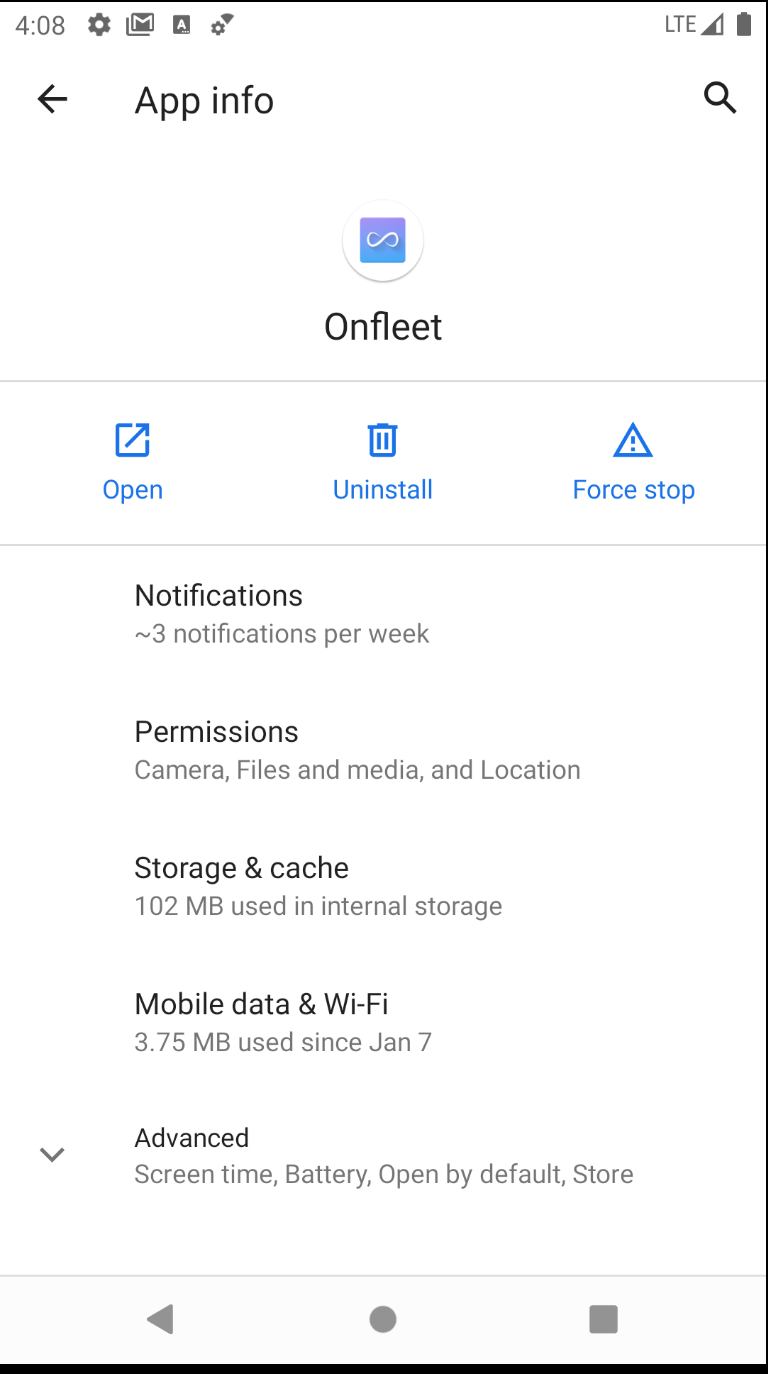In this image, a white smartphone is prominently displayed against a simple background, with the time indicated as 4:08 and an LTE signal visible. The screen features the "App Info" section for an application named "On Fleet." The app icon, a stylized sideways 'S', is positioned within a gradient blue box that transitions from light blue at the top to a brighter blue at the bottom. Below the app icon, options for "Open," "Uninstall," and "Force Stop" are clearly shown.

Further down, the screen displays several settings and data points related to the app. Notifications are set to three per week. Permissions granted include access to the camera, files and media, and location. The "Storage & Cache" section reports that 102 MB is used in internal storage, while "Mobile Data & Wi-Fi" indicates 3.75 MB of data used since January 7th. An advanced settings menu can be accessed via a down arrow, showing options like "Screen Time," "Battery," "Open by Default," and "Store." The interface is outlined in black, providing a neat frame around the detailed app information displayed on the screen. The bottom of the screen features three small icons, completing the layout.